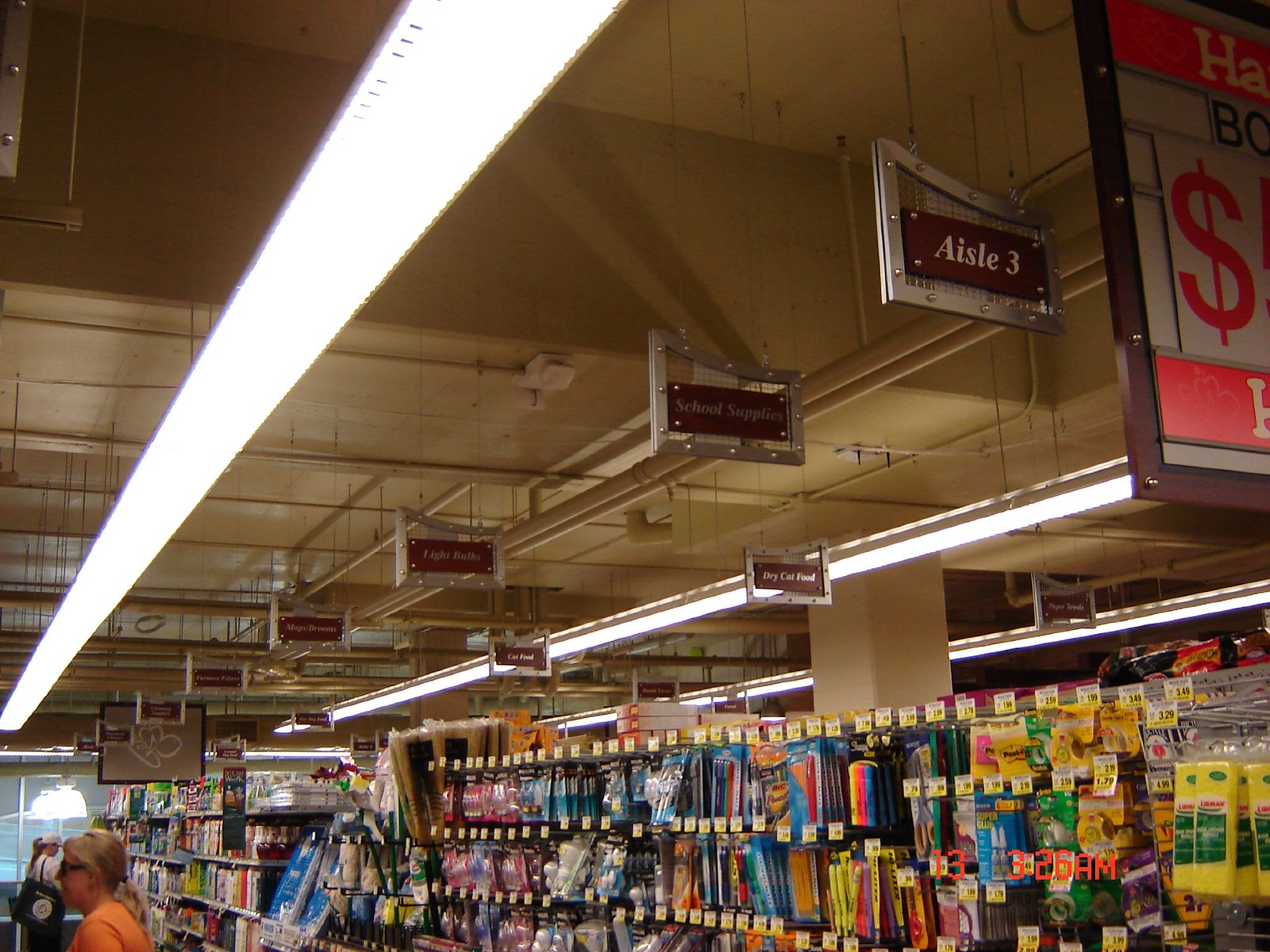This photo depicts the interior of a general store, characterized by its diverse selection of merchandise. The right side of the image prominently features a school supplies section, clearly identified by a suspended brown rectangular sign with a silver frame. The shelves below the sign display an assortment of packaged items including pens, pencils, highlighters, glue, and tape, each with white and yellow price tags. The scene is illuminated by natural daylight, contradicting the digital watermark in the bottom right corner that inaccurately reads "13" and "3:26 a.m." Additionally, a woman is visible within the frame, adding a human element to the busy retail environment.